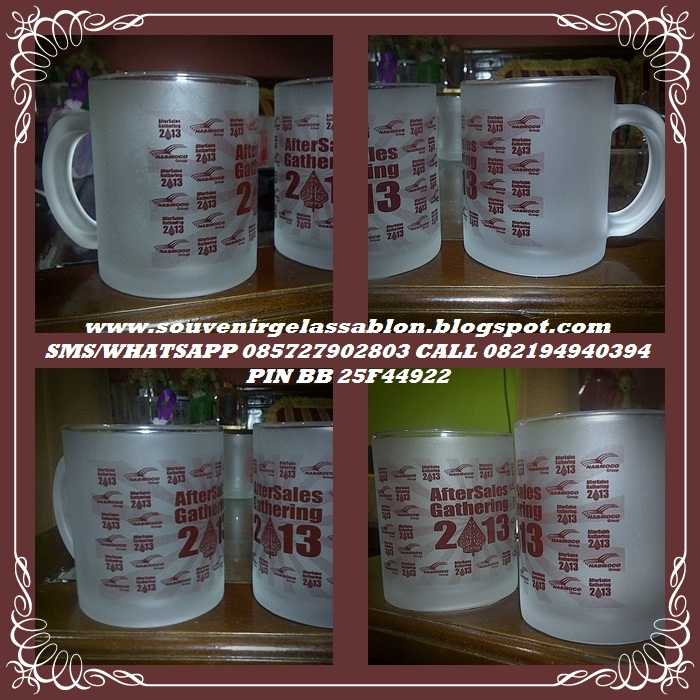The image presents a promotional advertisement for souvenir glass mugs intended for a magazine or similar publication. The central design features a square with a red pinstriped border, divided into four quadrants. Inside the quadrants, seven white frosted glass mugs are arranged, three on the top row and four on the bottom. Each mug bears red writing, displaying the phrase "After Sales Gathering 2013," with the "O" stylized as a Christmas tree. These mugs have U-shaped handles and are laid out against a light green background with a decorative white scroll design. Surrounding the arrangement, the borders are adorned with red squiggly, pinstripe patterns. In the middle section, the contact information is prominently displayed: "www.souvenirglassablon.blogspot.com, SMS/WhatsApp 085727902803, Call 082194940394, PIN BB25F44922", emphasizing both a visual and commercial element to attract potential buyers.